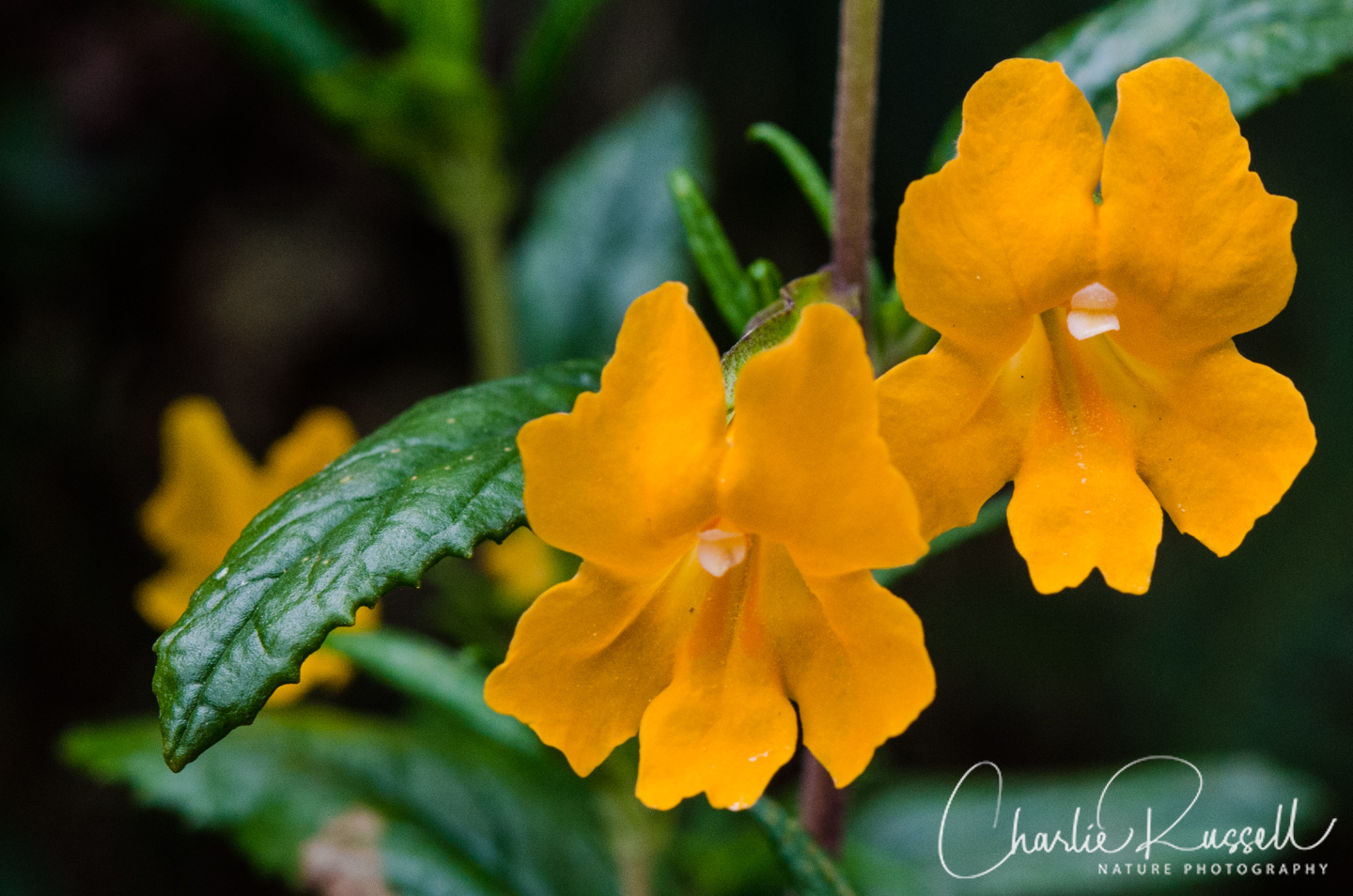This captivating photograph, titled "Charlie Russell, Nature Photography," showcases two bright yellow-orange flowers, both exhibiting five petals each—arranged with two at the top and three at the bottom. The primary flower is positioned prominently in the center, while the second flower is just above and slightly to the right. Each flower is accompanied by lush green leaves and a single stem, all brought into sharp focus.

The background of the image is deliberately blurred, highlighting the flowers and their leaves while providing a sense of depth with additional foliage and further blooms peeking through the darkness. The scene is set against a dramatic, almost black backdrop, creating a night-time ambiance and emphasizing the vivid colors of the blooms. 

In the lower right-hand corner, the photographer’s name, Charlie Russell, is elegantly inscribed in white script, with "Nature Photography" written in smaller print beneath. The photo, approximately 5 by 5 inches in size, encapsulates the serene beauty of nature with a detailed and intimate focus on the flowers.